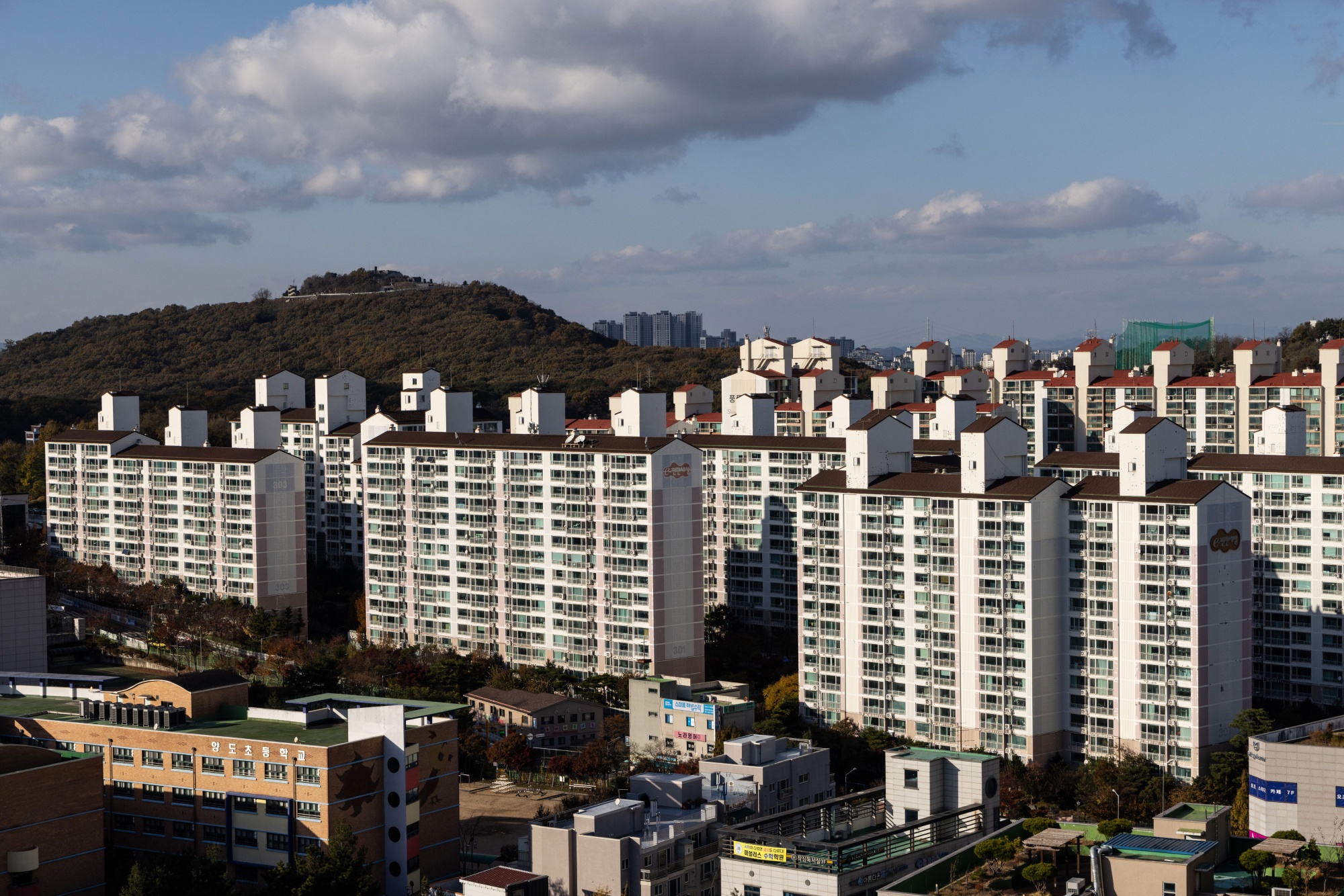The photograph captures a bustling cityscape dominated by tall, white-painted skyscrapers and high-rise apartment buildings arranged in rows. These imposing structures, with their multiple units and uniform white coloration, are front and center in the image. To the back right, some buildings stand out with distinctive red sloping rooftops. Closer to the ground, at the foot of these skyscrapers, smaller yet multi-storey buildings add to the urban density, displaying an array of grey and brown hues. On the left center side of the image, a verdant hill with lush trees provides a natural contrast to the man-made skyline. Above, the sky is a mix of blue and greyish tones, with clouds ranging from dark to white, setting a dynamic backdrop. The scene is clearly taken in daylight, emphasizing the architectural elements and the vibrant city atmosphere.